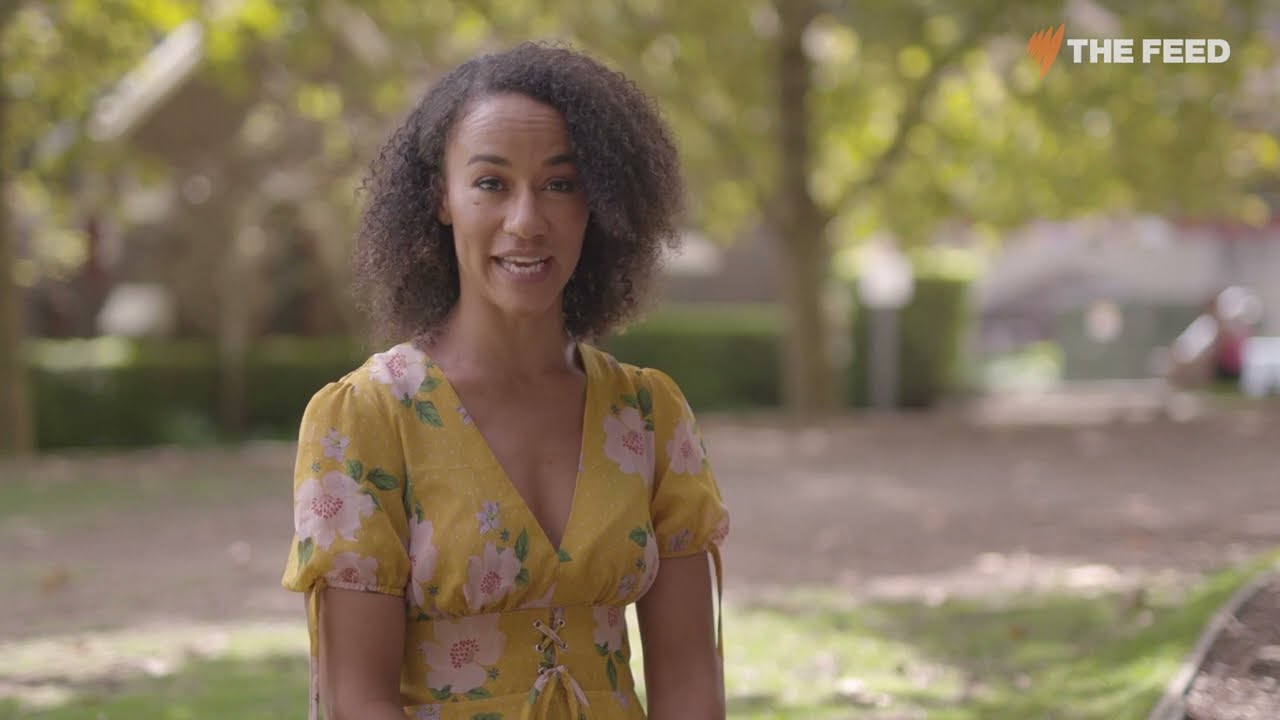The image captures a candid moment featuring an African-American woman, dressed in a bright yellow summer dress adorned with floral patterns, standing outdoors in a park. The woman, who has well-groomed, short, curly brunette hair, appears mid-speech, suggesting the image is a screenshot from a video. Her pose is natural rather than staged, reinforcing the idea of a live recording. Behind her, a backdrop of green trees and a hedge, partially blurred for an artistic effect, sets a serene scene typical of a professional production. To the right, a clearly visible walkway indicates the photo's outdoor setting during the day. In the upper right corner of the image, the logo "The Feed" in bold capital letters, accompanied by a yellow squiggle, confirms a possible association with a media company or a video uploader.